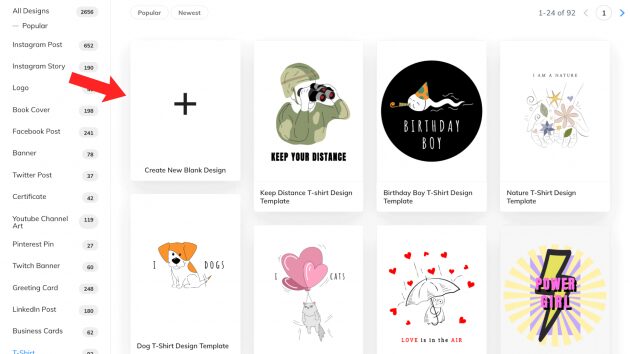The image features a detailed interface layout. At the top, the screen displays options labeled "Popular" and "Newest," with an indication that this is item one out of 24 of 92. On the left side, there is a sidebar listing various design categories, including "All Design," "Popular," "Instagram Post," "Instagram Story," "Logo," "Book Cover," "Facebook Post," "Banner," "Twitter Post," "Certificate," "YouTube Channel Art," "Pinterest Pin," "Twitch Banner," "Greeting Card," "LinkedIn Post," and "Business Cards."

To the right, a prominent square with a black plus sign in the middle features the text "Create New Blank Design" at the bottom. A red arrow points toward this square from the left side. Adjacent to it, on the right, there is another square displaying an image of a soldier in camouflage, looking through binoculars. This square includes the text "Keep Your Distance" and "Keep Distance T-Shirt Design Template" beneath it. Further to the right, another text reads "Birthday Boy T-Shirt Design."